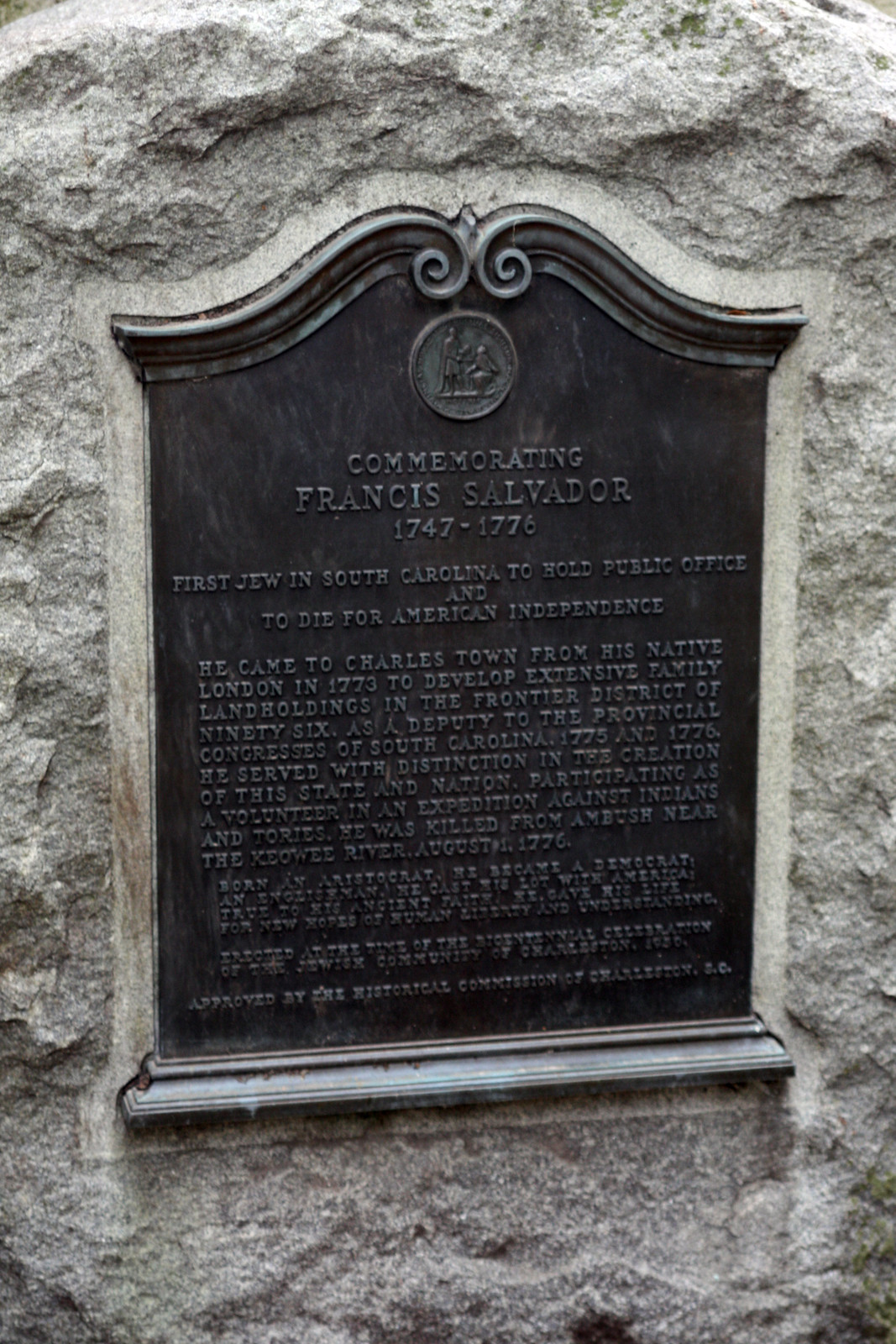The photograph, taken outdoors during the daytime, features a rectangular plaque set against a natural gray stone wall. The stone background, taller than it is wide, frames the plaque perfectly at its center. The metal plaque also mirrors the stone wall in its rectangular form, but with an artistic flair – its top edges rise upward in a wave-like arc, adorned with two curls and outward waves in the center.

At the top of the plaque is a circular engraving depicting a man standing while another kneels before him. Below this image, the main inscription is raised in black lettering against a slightly faded, almost gray-black surface. It reads: "Commemorating Francis Salvador 1747-1776. First Jew in South Carolina to hold public office and to die for American independence. He came to Charlestown from his native London in 1773 to develop extensive family land holding in the Frontier District of 96." Further text elaborates on Salvador's notable contributions: "As a deputy to the Provincial Congress of South Carolina in 1775 and 1776, he served with distinction in the creation of the state and nation, participating as a volunteer in an expedition against Indians and Tories. He was killed from ambush near the Keowee River, August 1776."

The smaller, more intricate text toward the bottom adds: "Born an aristocrat, he became a Democrat. An Englishman, he cast his lot with America. True to his ancient faith, he gave his life for new hopes of human liberty and understanding." The plaque concludes by noting its erection during the bicentennial celebration of the Jewish community of Charleston in 1930, with the approval of the Historical Commission of Charleston, South Carolina. The overall setting and text suggest a solemn tribute, potentially located in a cemetery or memorial site.